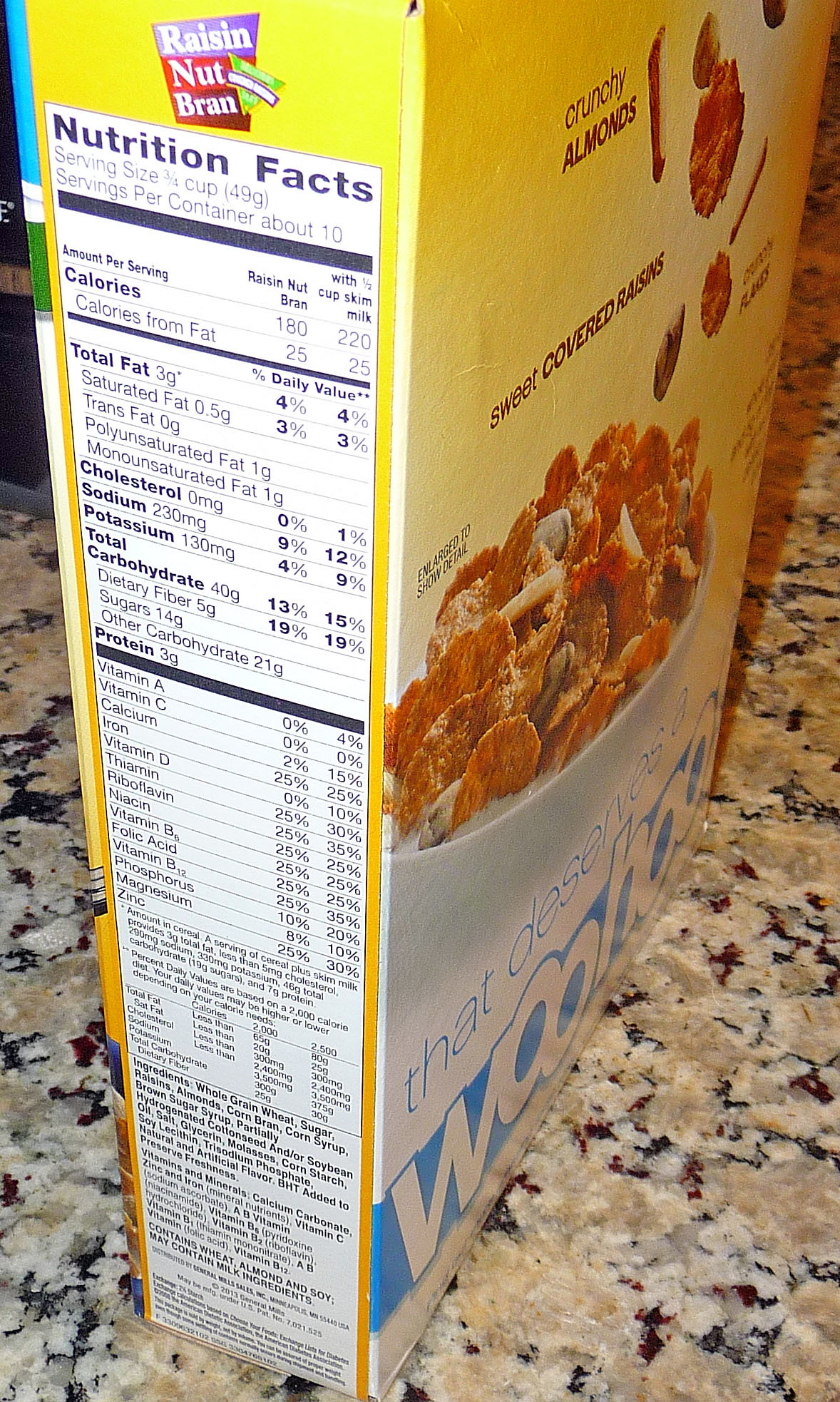The image captures a Raisin Nut Bran cereal box resting on a sophisticated granite countertop, characterized by its distinctive tan, dark brown, and black splotchy pattern. The focal point of the image is the nutrition label positioned towards the camera, albeit slightly angled to the left. Consequently, the rear section of the box is partly visible on the right-hand side. The prominently displayed Nutrition Facts section at the top of the label, although somewhat difficult to read in detail, features the standard nutritional and ingredient information found on most American food packaging.

The front of the cereal box showcases a vivid depiction of a white bowl brimming with cereal flakes, crunchy nuts, and succulent raisins. Above the bowl, various cereal pieces appear to be cascading downwards, adding a dynamic touch to the design. The box itself predominantly features a bright yellow background, enhancing the visual appeal and making it instantly recognizable on any shelf.